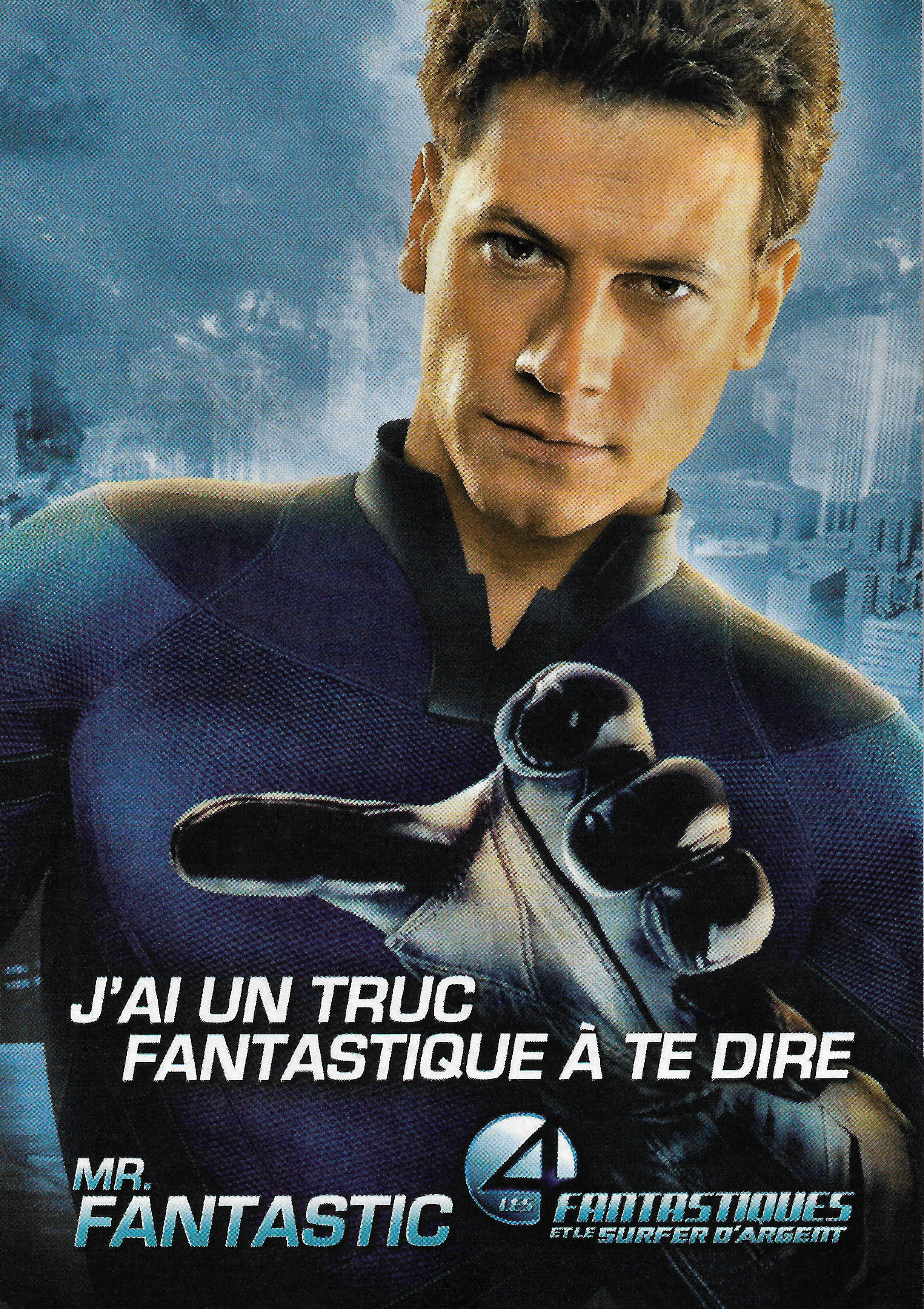The image is a poster for the Spanish or French version of the movie *Fantastic Four: Rise of the Silver Surfer*. The central figure is Mr. Fantastic, depicted by a young actor, wearing a form-fitting blue suit with black leather gloves. His left arm is stretched out towards the viewer, looking as though he's about to grasp something. The background showcases a blue cityscape, possibly with elements that resemble crystals or ice. The text on the poster includes "J'ai un truc fantastique à te dire" in white letters, and beneath it, "Mr. Fantastic" in blue capital letters. The bottom right of the poster features the title "Fantastic Four: Silver Surfer" in French or Spanish. The overall color scheme includes shades of blue, black, tan, brown, and white. The layout places Mr. Fantastic diagonally across the poster, with his head tilted to the upper right corner.